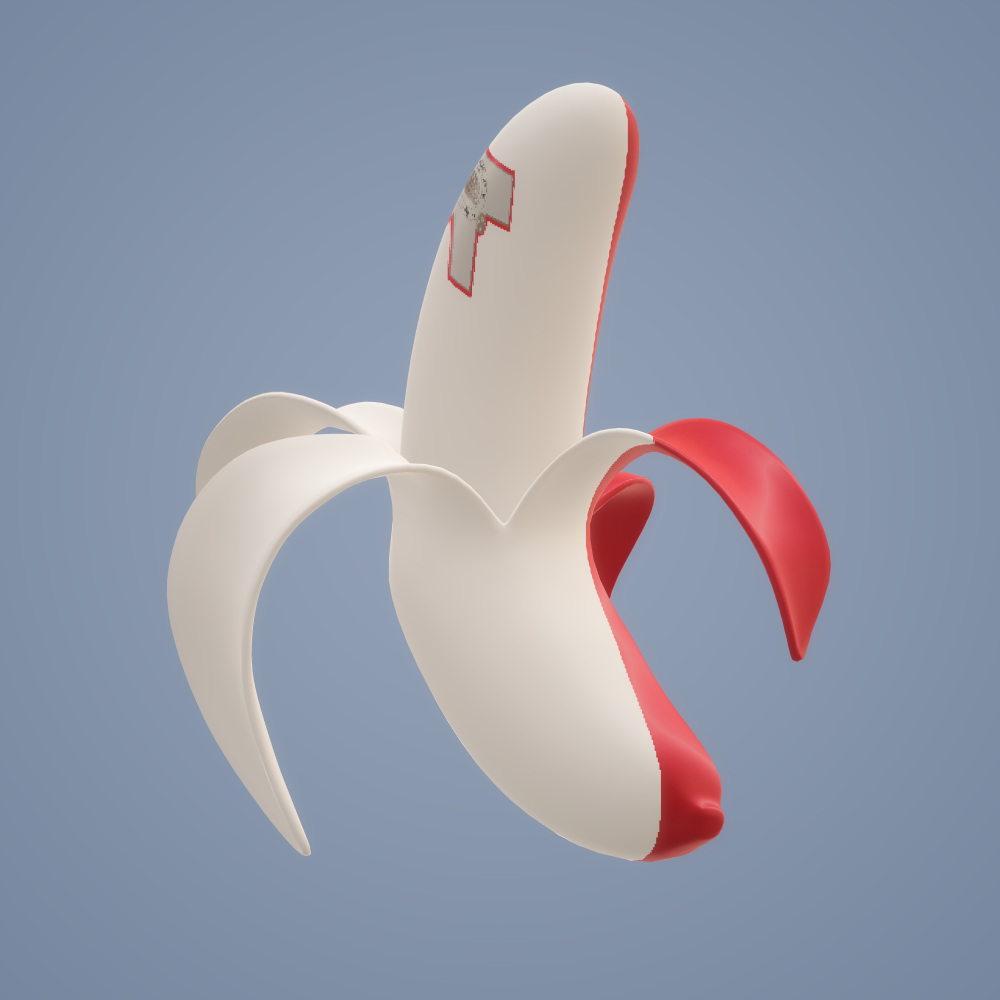The image likely depicts a 3D-rendered, non-edible banana with a vinyl-like texture, set against a dark bluish-gray background that is highlighted in the center and fades to darker shades at the corners. The banana is split into a red and white color scheme, running lengthwise. It is partially peeled into four sections—two red and two white. The fruit itself follows the same color division; predominantly white on the visible front side and red on the back side. The white portion of the banana features a gray logo outlined in red, resembling the letter 'T'. The banana and its peel appear artificial, possibly made of vinyl or designed as a symbolic object or perhaps a dog toy.